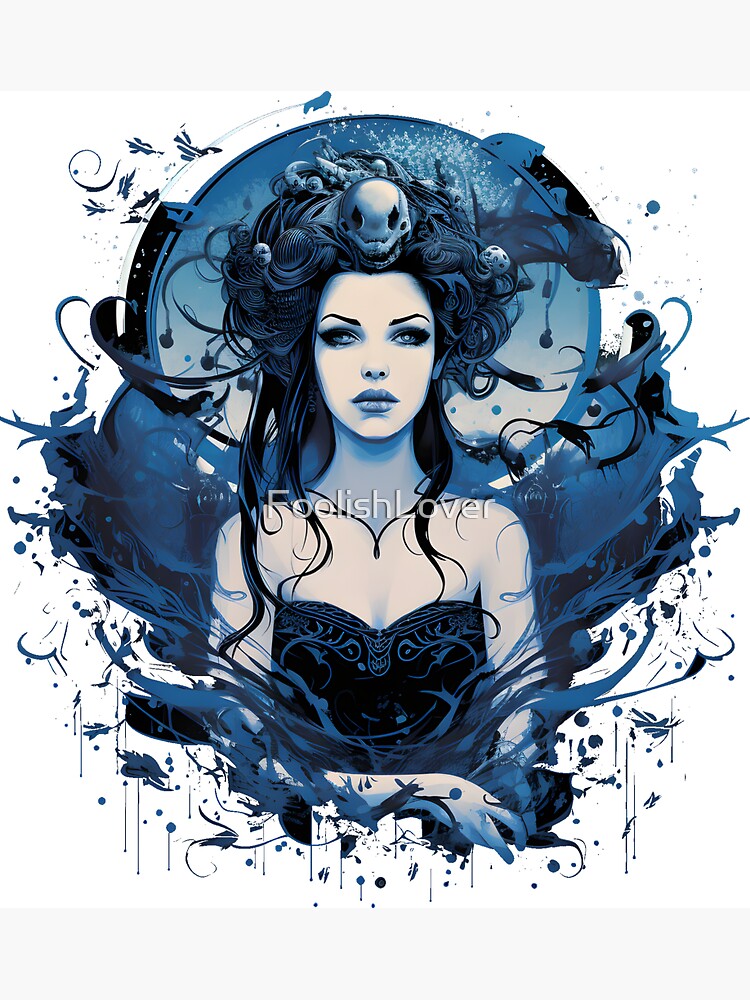The image is a detailed artwork, primarily rendered in varying gradients of blue ink, giving it a cohesive and striking monochromatic palette. At the center of this piece, there is a watermark or caption that reads "Foolish Lover" in capital letters, specifically rendered as "F-O-O-L-I-S-H L-O-V-E-R". It depicts a woman, visible from the waist up, with her arms folded at her midsection and hands partially visible. She wears a dark, strapless top, possibly a tank top or halter style, adorned with a subtle blue design inside it. The woman has lighter skin with a bluish tint, complemented by blue eyes and blue lips, and intense black eyeliner accentuating her gaze.

Atop her head, she wears a distinctive headdress that resembles a skull, entwined with strands of hair-like elements that swirl around it. Her voluminous black hair is styled in chaotic, flowing directions, adding to her enigmatic appearance. Surrounding her is a circular gradient of blue, and watery, paint-like splashes extend from her arms and the background, creating a dynamic and fluid effect. The overall tone of the artwork is serious and slightly demonic, with the intricate blue shades and splashes enhancing its ethereal, hauntingly beautiful quality.